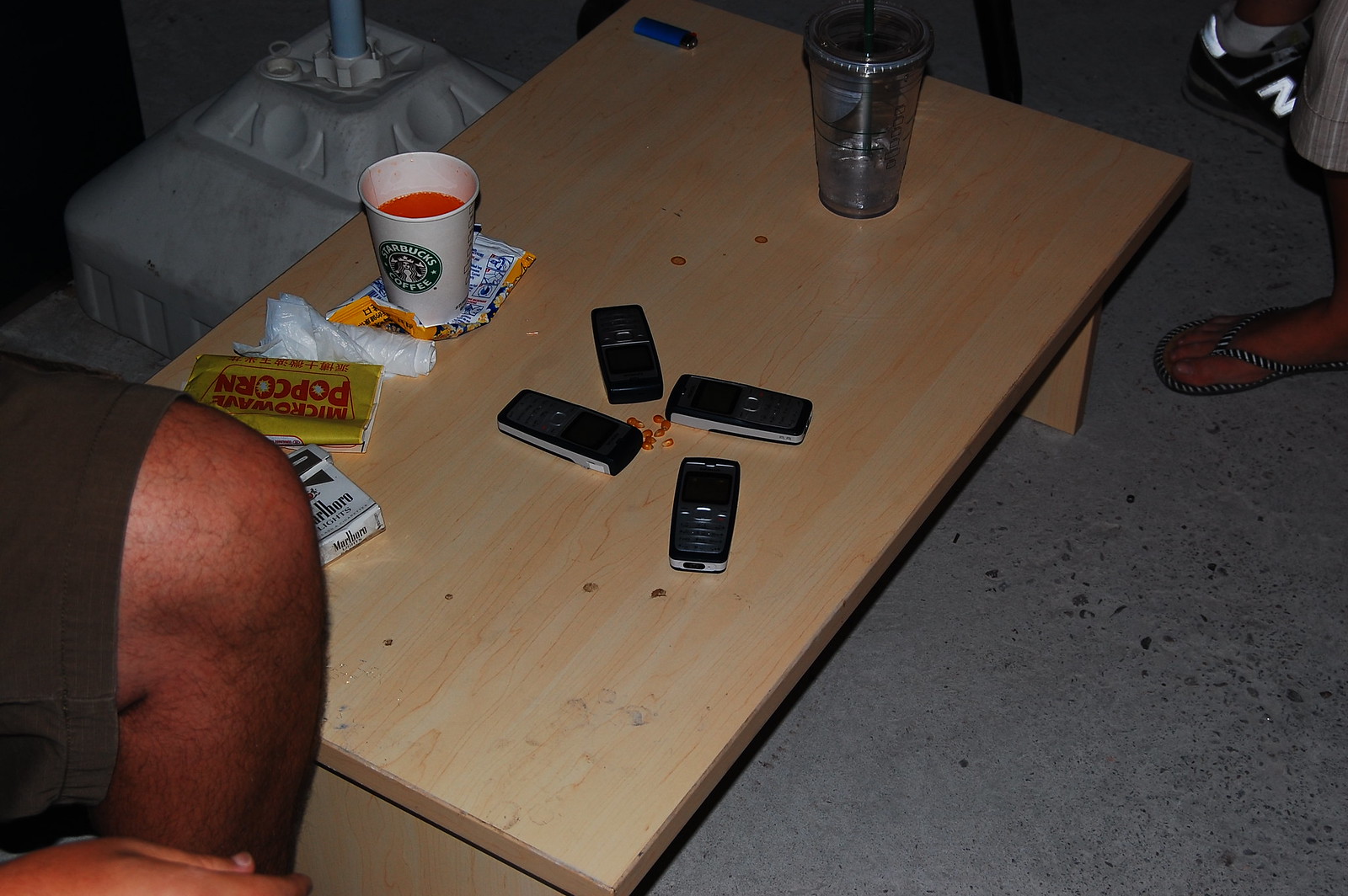This image depicts a scene centered around a light-colored wooden coffee table cluttered with various items. Dominating the tabletop is a plastic iced coffee cup, seemingly empty, accompanied by a blue lighter. At the heart of the table, four older-style black cell phones are arranged in a circle, their tops facing inward. In the middle of these phones lie some pretzel bits. Nearby, a Starbucks cup containing a red liquid is precariously balanced atop a small bag of chips, turned upside down. Adjacent to this setup is a microwave popcorn bag and a pack of Marlboro cigarettes positioned at the table's corner. Framed on the left side of the image, partially seen, are a man's legs wearing shorts, while on the right, another person’s foot donned in a flip-flop sandal is visible, along with a distant shoe bearing an "N" logo. The table sits on a gray floor, contributing to the room's overall dim ambiance, enhanced by the presence of a whitish-gray object base on the left side.